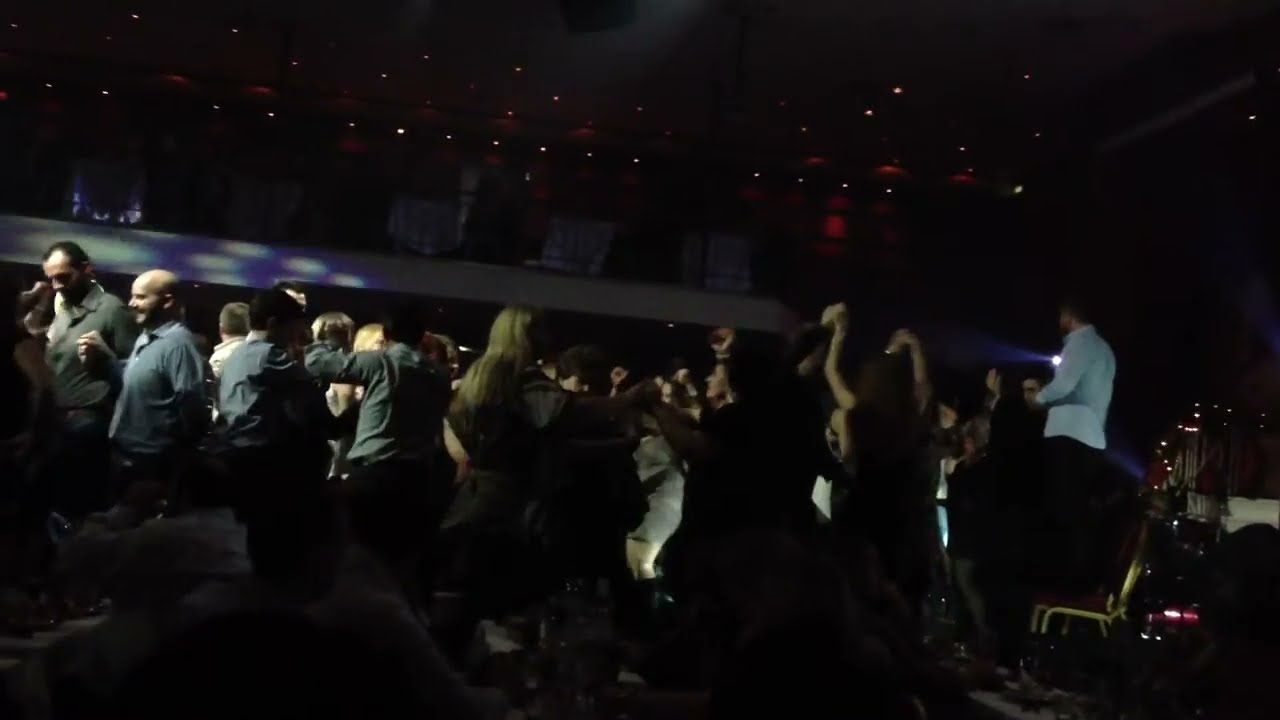This full-color photograph captures a lively indoor scene at what appears to be a dimly lit party hall, possibly a bar, nightclub, or hotel ballroom during an event. The space is buzzing with activity, dominated by a crowd of adults, both men and women, who are dancing and socializing. The men are dressed in business casual attire, while the women appear to be wearing dresses. Most of the light is focused on the central dance floor, highlighting the energetic dancers with raised arms, suggesting a joyful atmosphere. Overhead, a mix of red and white lights casts a subdued glow, barely illuminating the seated guests at tables on the periphery. The photograph also reveals a second level with more tables covered in white cloths and additional white lights, though these tables seem to be unoccupied. A stage area is present, albeit not clearly visible, with a person dressed in a blue shirt slightly elevated, possibly indicating a performer or musician. A solitary empty chair is noticeable at the lower right of the image, adding to the intricate details of this bustling, yet somewhat darkly lit party setting.